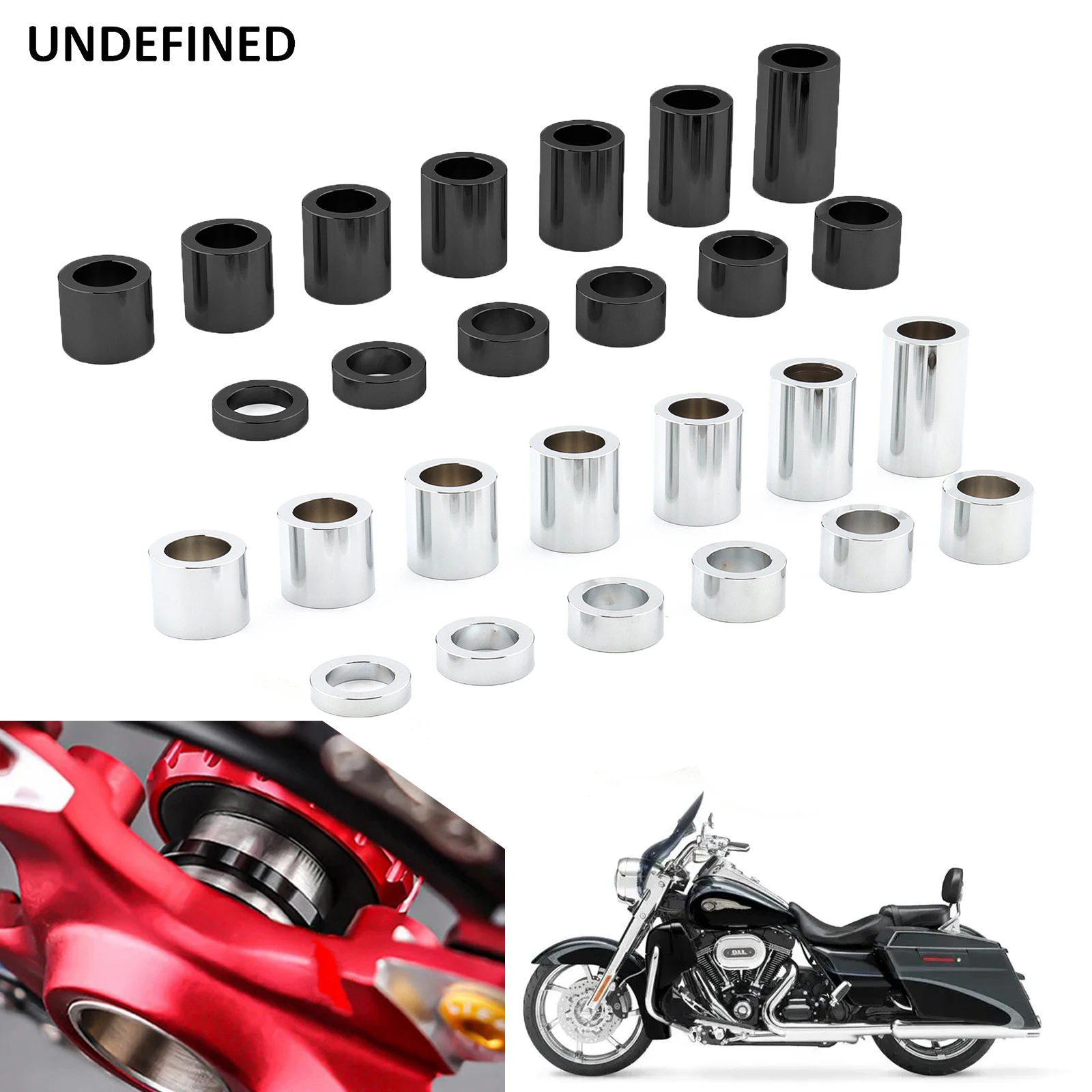The image displays a detailed layout of motorcycle parts against a white background, with the caption "UNDEFINED" in black capital letters at the top left. Central to the image are four diagonal rows of cylindrical metallic components resembling axle spacers or similar fittings, positioned from bottom left to top right. The first two rows feature shiny black spacers, arranged from shortest to tallest from left to right. Below them, the next two rows display similar components in silver, following the same height arrangement. At the bottom left of the image, there is a close-up of a red motorcycle part, suggesting where these cylindrical pieces might be installed. The bottom right corner showcases a cruiser-style black motorcycle with silver trim, facing left. The overall setting is well-lit, highlighting the metallic sheen and details of the components.